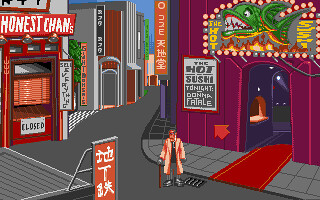This image depicts a scene from a retro-style, 8-bit video game reminiscent of early Nintendo or Sega classics. The low-resolution graphics evoke a sense of nostalgia, featuring a bustling city street lined with various storefronts. Notable businesses include "Honest Chan's" and "The Hot Sushi," alongside a distinctive nightclub adorned with a purple facade and a green fish emblem. At the center of the screen stands a figure, likely the playable character, dressed in a brown trench coat. The overall atmosphere captures the vibrant yet pixelated aesthetic typical of vintage video games.